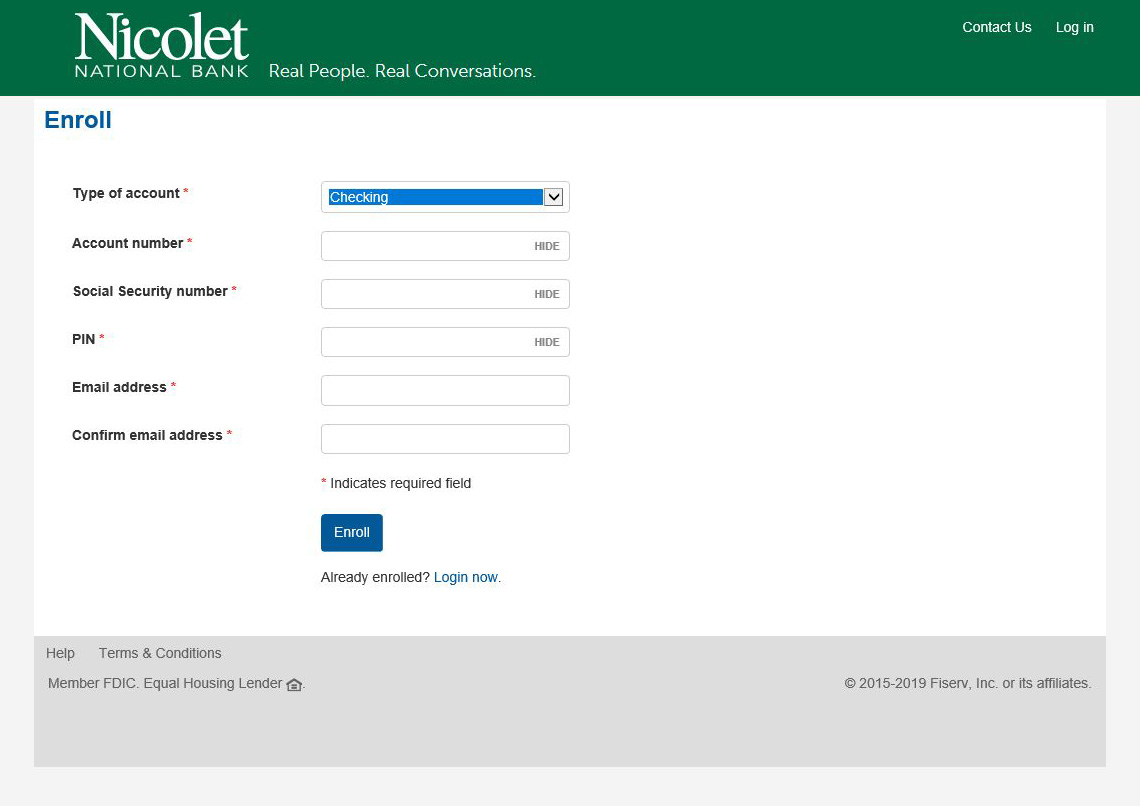The image depicts the website interface for Nicollet National Bank, prominently showcasing the bank’s name in the top left corner, set against a green panel. On this same panel, located in the upper right, are clickable links for "Contact Us" and "Login."

Underneath this heading, the main section features a predominantly white screen. Along the left-hand side is a blue "Enroll" heading followed by a series of input labels and fields for new user enrollment. These include:

1. **Type of Account**: A dropdown list currently displaying "Checking" in blue.
2. **Account Number**: An empty input field with an adjacent "Hide" button for confidentiality.
3. **Social Security Number**: Another empty input field, also with a "Hide" button.
4. **PIN**: Similarly, an empty input field with an option to hide the entry.
5. **Email Address**: An empty input field meant to capture the user’s email.
6. **Confirm Email Address**: Another empty input field to confirm the email provided above.

Each of these fields is marked as required, indicated by an asterisk or other visual cue on the screen. At the bottom of these input fields is a prominent blue "Enroll" button, which users can click to submit their information and begin the enrollment process.

For users who already have an account, there's a separate "Login Now" button situated just underneath the "Enroll" button. The bottom of the screen features a grey panel containing general terms and conditions along with help information.